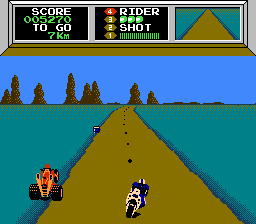The image is a still from a racing video game featuring two players. One player is riding a white motorcycle, and their character is colored deep blue. The other player is on an ATV, distinguished by its thick tires at the back, and their vehicle is yellow and red. They are racing on a road flanked by dull green areas, possibly representing grass, although not rendered in high detail. The background includes a few trees, adding some elements of nature to the setting. The game's interface shows a score of "005270" and indicates 7 kilometers left to go. Additional text on the screen includes "Rider" and "Shot," suggesting a possible gameplay mechanic involving shooting, though its exact function is unclear from the still image.